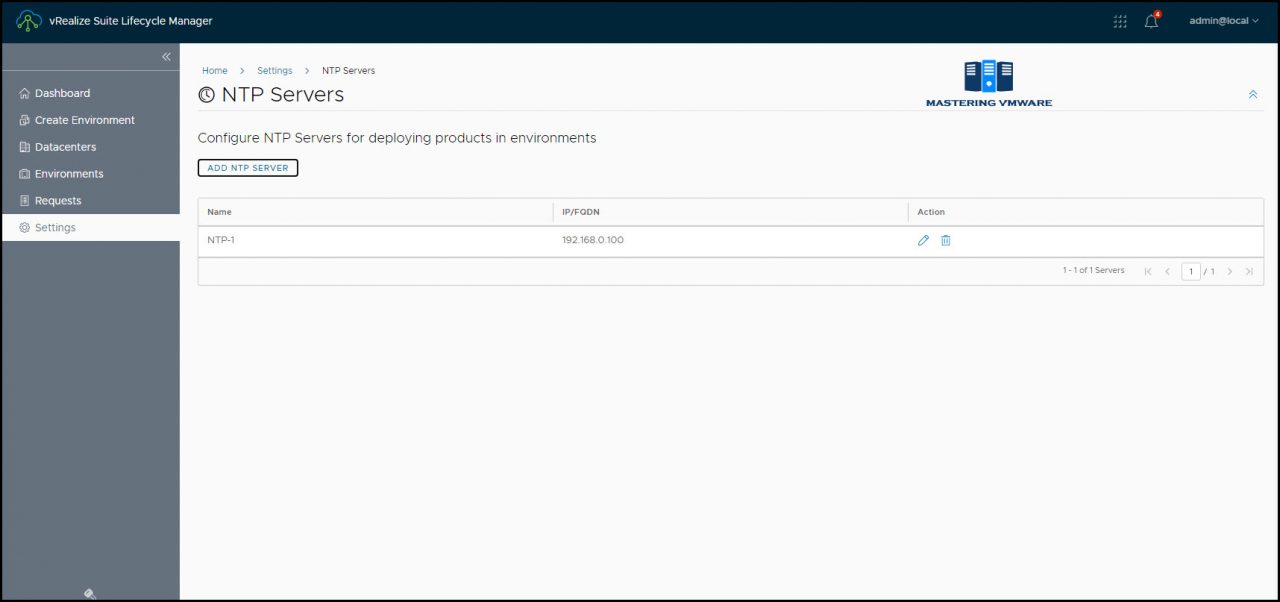The screenshot captures a web page titled "Something Sweet, Lifeguard Manager." At the top, the title bar is slightly blurry but readable. A vertical navigation menu is located on the left side of the page, featuring options such as "Dashboard," "Create Environment," "Data Centers," "Environments," "Requests," and "Settings," with "Settings" being highlighted in white text on a blue background, indicating its current selection.

The main content area of the page is dedicated to the configuration of NTP servers. The heading "NTP Servers" is prominently displayed, with a subheading that reads, "Configure NTP servers for deploying products in environments." Below this, there is a button labeled "Add an NTP Server."

A table is visible beneath the button, containing a single entry. The table columns include "Name," "Purpose or Program," "IP Address," and "Action." The entry shows the NTP server named "NTP-1," an unclear purpose or program (indicated by the text being difficult to read), and an IP address: "192.168.0.100." The action column includes a pencil icon for editing and another icon for additional actions.

In the upper right corner of the page, there is a label "Mastering View Name" with an icon resembling a library, suggesting it is clickable for more information.

Overall, the image presents a detailed view of the NTP server configuration section within a web application, highlighting the user interface elements and the current state of the page.